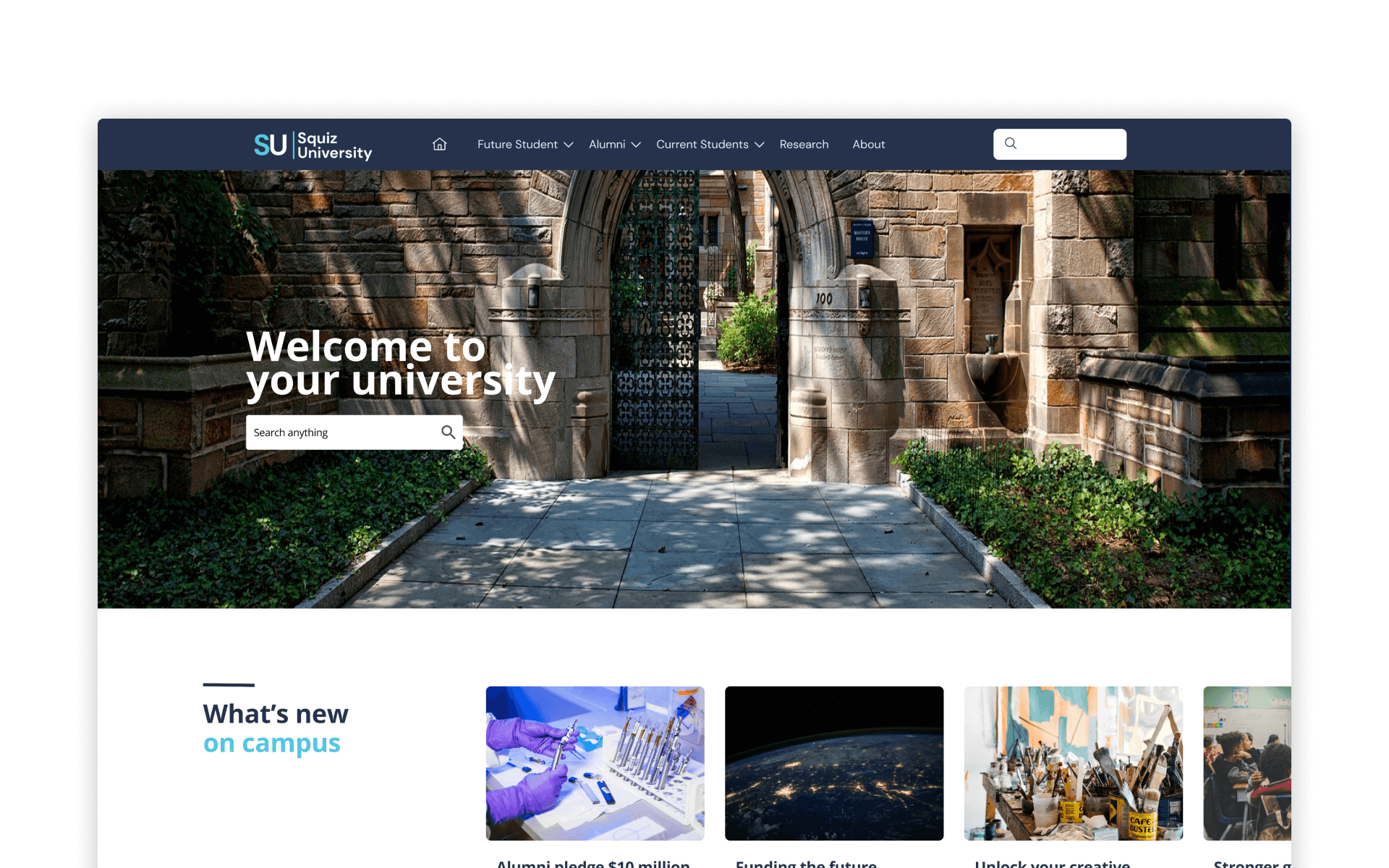The image depicts the homepage of the SQUIZ University website. At the top of the page, there is a dark blue navigation bar featuring pull-down menus labeled "Future Students," "Alumni," "Current Students," "Research," and "About." Adjacent to these menus, a prominent "SU" logo sits next to the full name "SQUIZ University."

Below the navigation bar, the main section welcomes visitors with a bold message: "Welcome to Your University." A search bar is conveniently positioned to allow easy access to further information.

The lower half of the webpage showcases a carousel of announcements titled "What's New on Campus." This section highlights updates such as "Alumni Pledge $10 Million," "Funding the Future," "Unlock Your Creative Potential," and "Stay Strong." However, the text appears partially obscured as it scrolls.

The central image on the page is a majestic view of the university's architecture. Dominating the scene is a grand stone brick wall, accentuated by an elegant archway. The arch frames an intricate black wrought iron door, resembling lace panels. Ivy decorates the foreground, accompanied by a tree casting dappled sunlight over the entrance. The gate stands open, with the inscription "Welcome to Your University" clearly visible, inviting visitors to explore further.